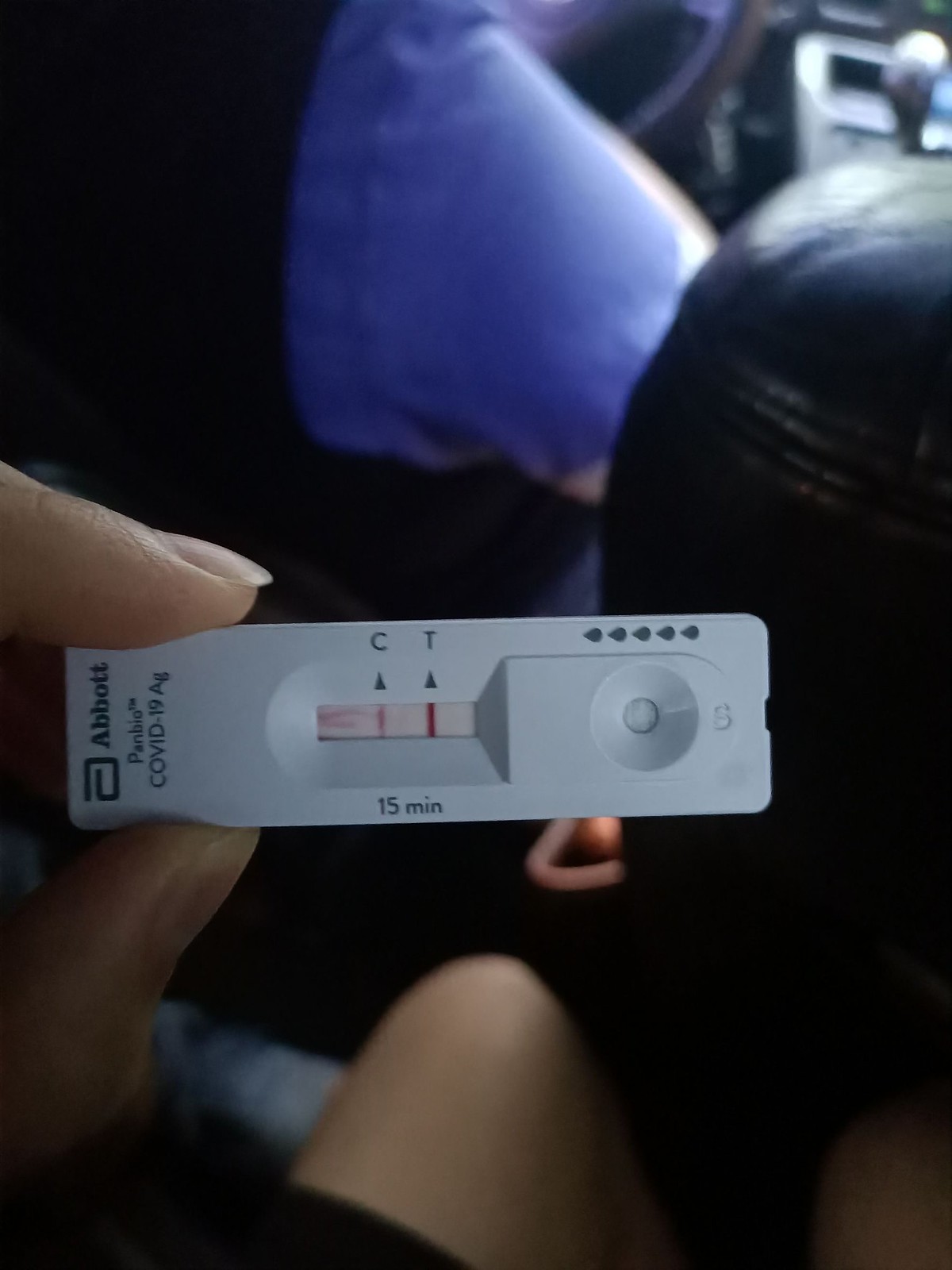In this close-up photograph, a Caucasian female's left hand is prominently featured, delicately holding a COVID-19 test device between her thumb and index finger. Her left knee is clearly visible, while her right knee is mostly cropped out of the frame, subtly indicating her seated position. The test, which appears light gray due to shadowing but is likely white, is labeled "Abbott" at the top, followed by "PanBio™" and "COVID-19 AG." Below these labels, it notes "15 minutes." The test strip shows two indicators labeled ‘C’ and ‘T’ above arrows that point to the respective result lines. Notably, the ‘C’ line on the right is bold and vivid red, whereas the ‘T’ line on the left is faint and barely discernible.